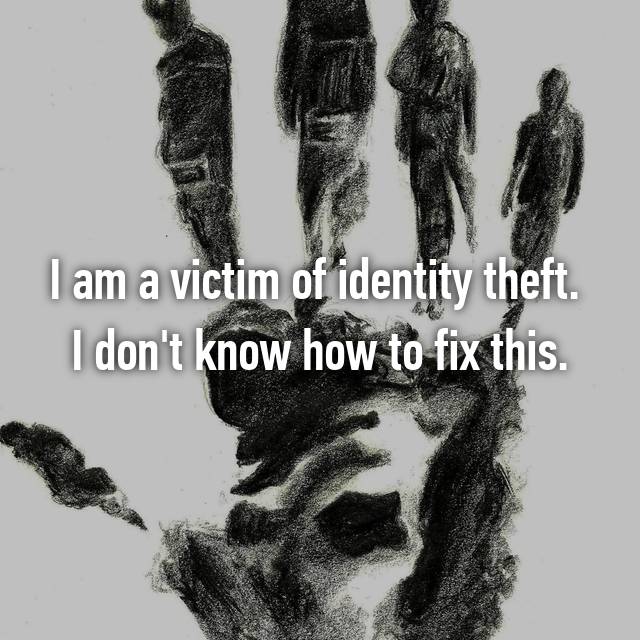The graphic features a light gray background with a compelling charcoal drawing at the top, depicting the backs of four human figures whose identities blend ambiguously into one another, forming a chaotic mix of overlapping shadows. The bottom half of the artwork continues this theme of disarray, with their shadows jumbled together, creating an abstract and confusing pattern that symbolizes the entangled mess of identity theft. In the center of the image, two rows of white text read, "I am a victim of identity theft. I don't know how to fix this," underscoring the confusion and hopelessness of losing one's identity. The entire piece collectively portrays the disorienting and unsettling experience of identity theft, with a unique artistic representation that combines human silhouettes and abstract forms to vividly convey the emotional turmoil involved.